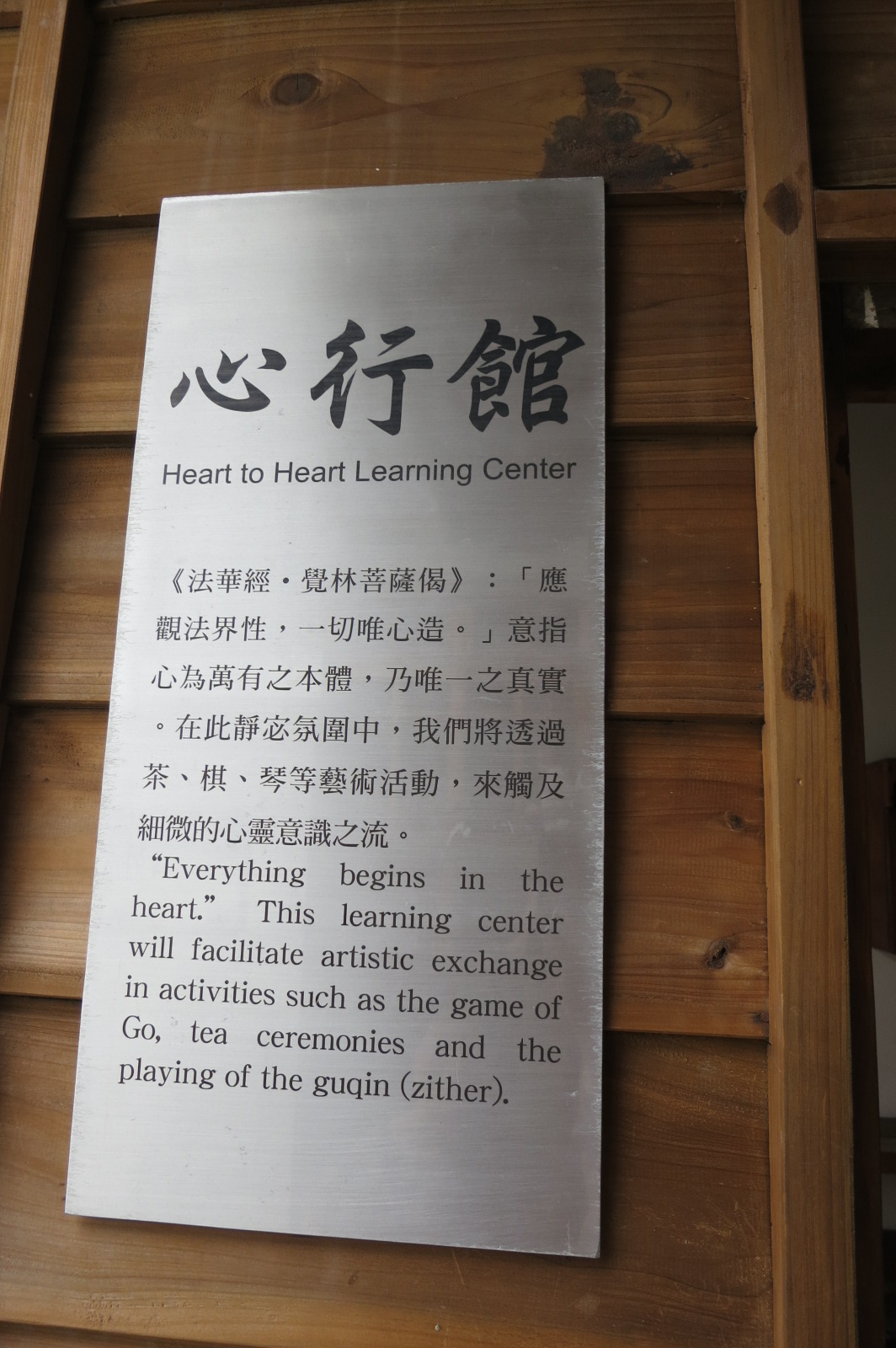A silver metal plaque is mounted on a wooden wall featuring paneling or slats. At the top of the plaque are three large Chinese or Japanese characters, likely Japanese. Beneath these characters, an English translation reads, "Heart-to-Heart Learning Center." Further down, there's a passage written first in smaller Chinese or Japanese text, which is then translated to English as, "Everything begins in the heart." The plaque states that the learning center aims to facilitate artistic exchange through activities such as the game of Go, tea ceremonies, and the playing of the Guqin, with "zither" noted in parentheses. The plaque is positioned next to what appears to be a doorframe, although the doorframe is only partially visible in the image.